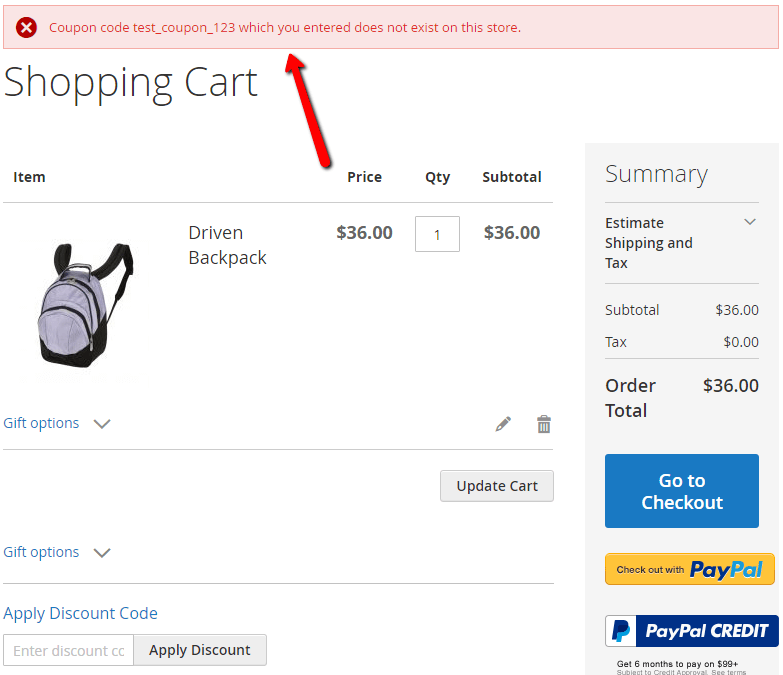This image is a cropped and enlarged screenshot of a shopping cart on an e-commerce website. At the top of the image, a red banner spans the width of the screen, featuring a red rectangle with a white "X" on the left, and red text to the right stating: "Coupon code testcoupon123 which you entered does not exist on this store." A red arrow has been edited onto the screenshot, pointing directly at the error message, located in the center of the screen and pointing upwards.

Below this alert, on the left side, the section is titled "Shopping Cart" in large black letters. Beneath the title, there is a thumbnail of an item labeled "Driven Backpack." Above the item thumbnail are the headings: "Item," "Price," "Quantity," and "Subtotal." Specifically, the price is listed as $36, the quantity is set to 1, and the subtotal is also displayed as $36. Adjacent to the item thumbnail, "Gift options" is written in blue text with a dropdown box next to it. To the right of the gift options are a pencil icon (likely for editing) and a trash can icon (likely for deletion). At the bottom right, there are buttons labeled "Add to Cart" or "Update Cart," an "Apply Discount Code" textbox, and a gift options dropdown box.

On the right side of the image, a gray panel runs vertically down the page, displaying a summary of the order. At the top of the panel, it reads "Summary" followed by sections for "Estimate Shipping and Tax," "Subtotal," "Tax," and finally the "Order Total" at the bottom. A prominent blue box labeled "Go to Checkout" is located just above two PayPal options: "Checkout with PayPal" in yellow and "PayPal Credit" in blue.

This detailed layout provides a comprehensive overview of the shopping cart, error message, item details, and checkout options on the e-commerce website.